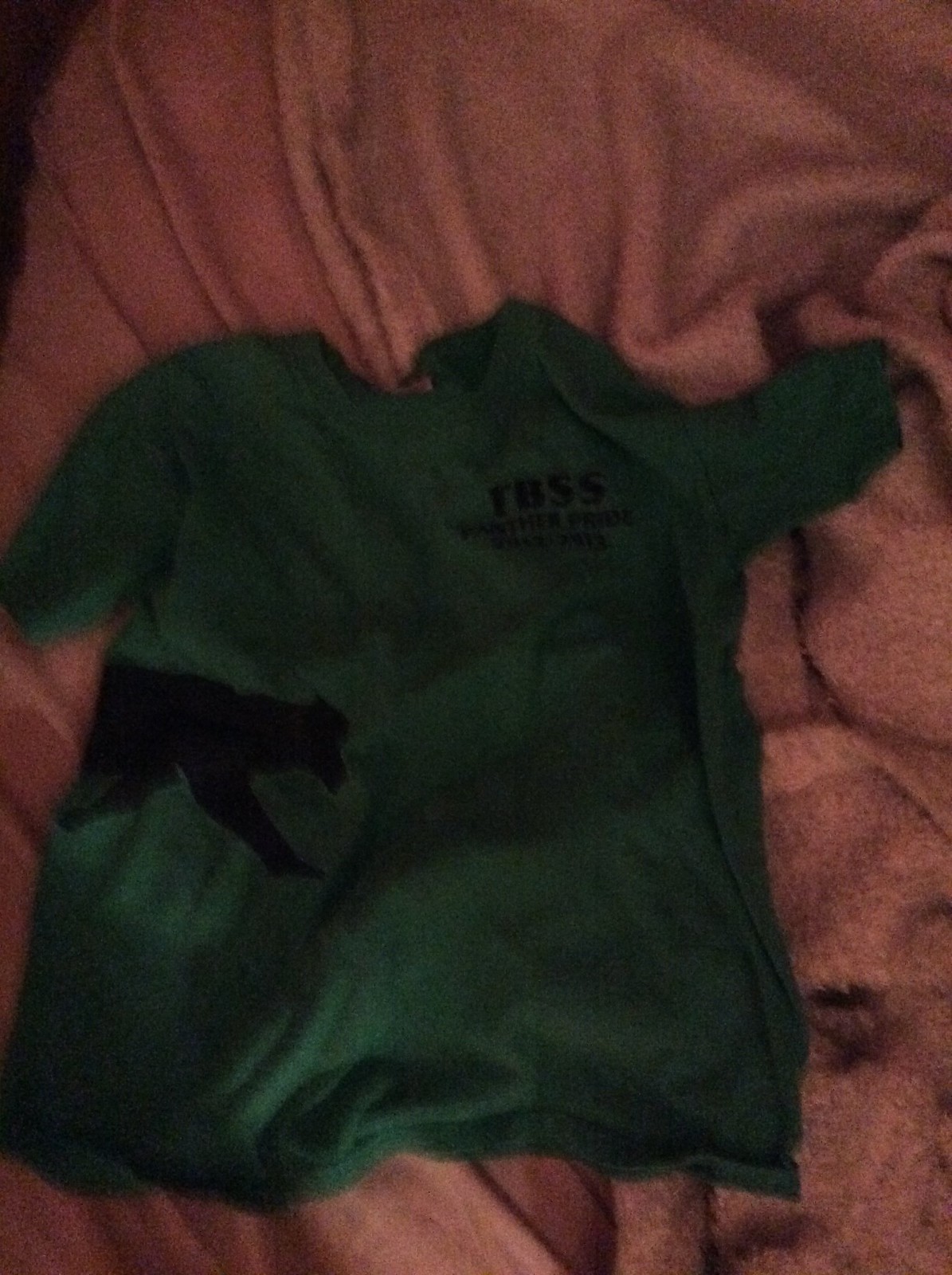A grainy and dark photograph, likely captured indoors using natural light, depicts a green short-sleeved, round-necked top laid out on a rose-pink blanket. The blanket's fabric is textured with numerous folds, ridges, and valleys. The green top, which appears to be made from a soft, thick material, features black lettering on the chest pocket area. Despite the blurriness, the contrasting colors and textures of the top and blanket create a visually interesting composition.